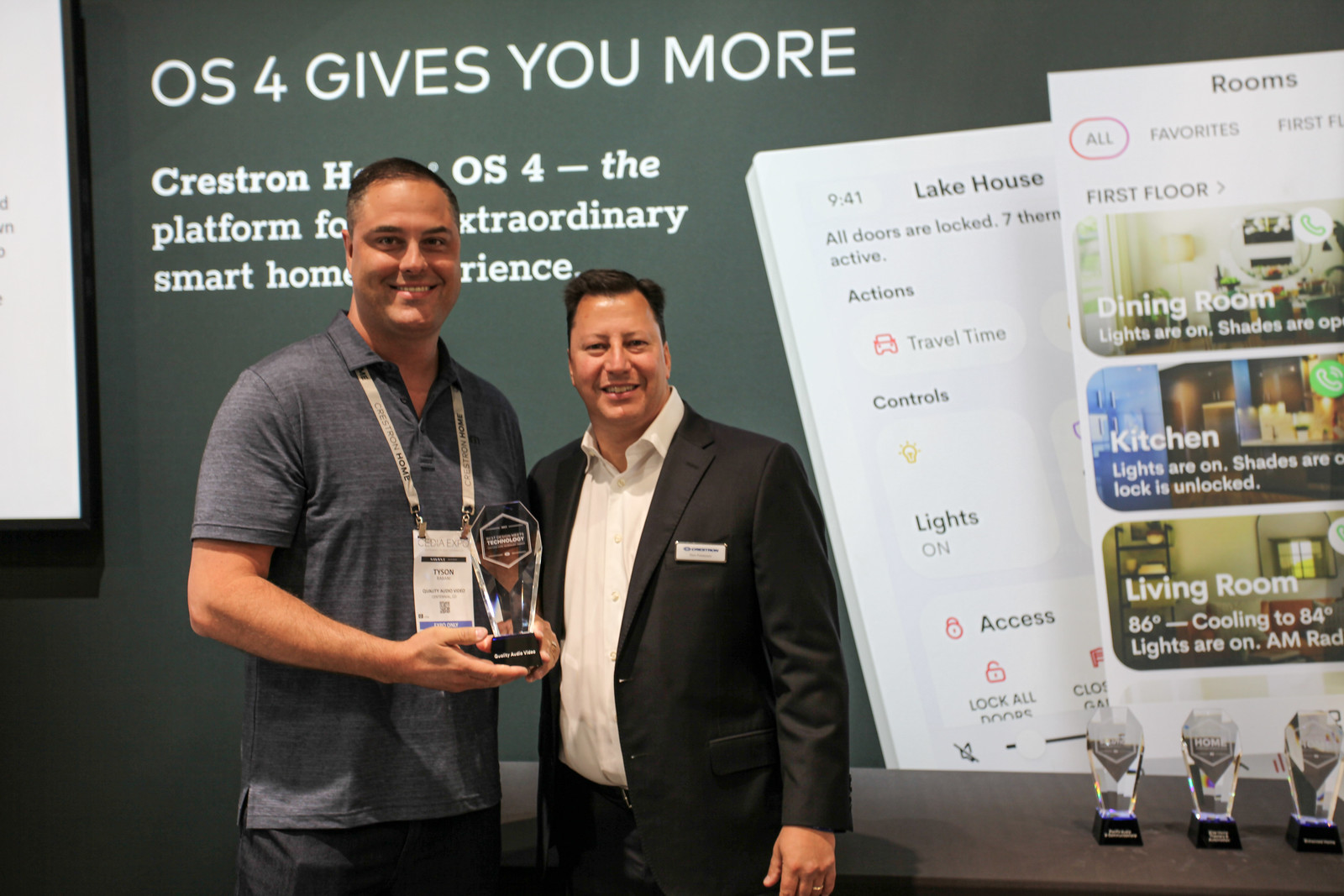The image captures an award ceremony where two men are standing in front of a sage-green backdrop emblazoned with white text that reads "OS4 gives you more," and partially obscured additional text including the word "Crestron." The backdrop features images and text detailing the capabilities of the OS4 platform, highlighting its control over smart home functions for areas such as the dining room, kitchen, and living room.

On the left stands a tall gentleman, smiling at the camera, wearing a white lanyard around his neck, and holding the award he has just received. To his right, a shorter man in a black suit and white shirt without a tie is presenting the award, also smiling at the camera. 

In front of them, there is a table displaying three clear trophies. The backdrop also includes illustrations emphasizing features like locking all doors and managing the house's lighting and room settings. The ambiance suggests a formal event celebrating technological innovations in smart home solutions.